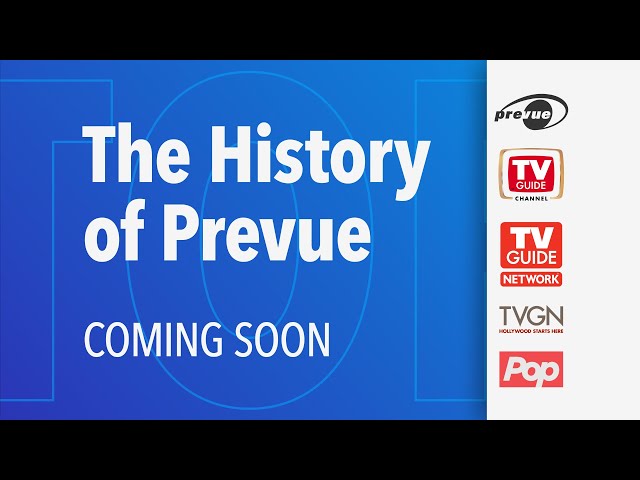This image appears to be a screen capture likely showcasing a thumbnail for an upcoming video or television segment. The screen features a blue background with white text prominently displayed in the center that reads, "The History of Preview: Coming Soon." To the right of the text, there is a vertical white box containing various logos and titles in sequential order: "Preview," represented with a logo resembling a human eye, followed by "TV Guide Channel," "TV Guide Network," "TVGN," and "Pop," along with the tagline "Hollywood Starts Here." The image seems to hint at a documentary or informative piece about the evolution and role of television guide services, specifically focusing on the Preview Channel and its transformation into TV Guide Channel and subsequent iterations.